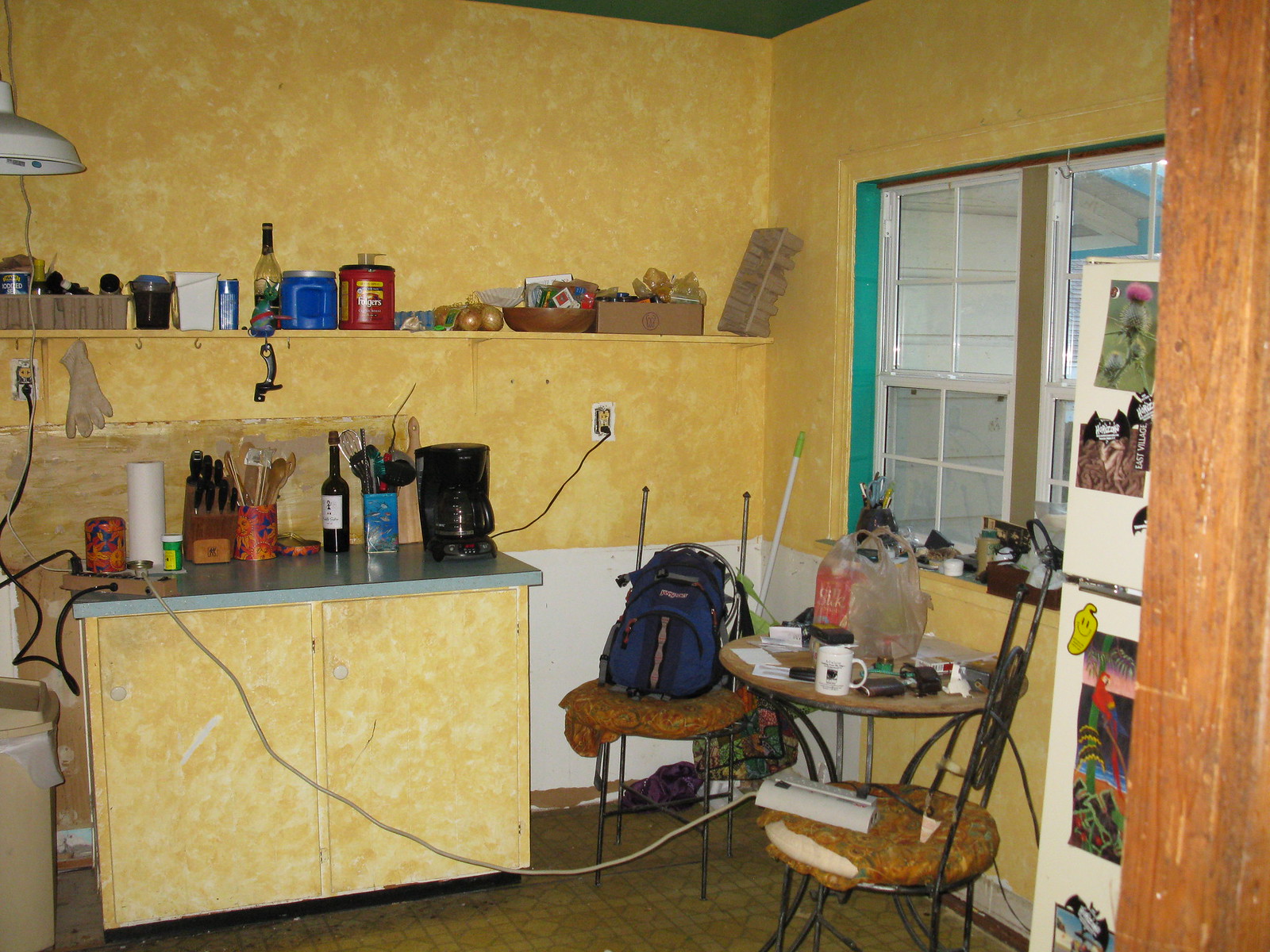The photograph captures a cluttered and haphazardly organized room. Dominating the visual space is a wall constructed from plywood or painted a yellow hue, intersecting the room. A window is set into this wall, framed by distinctive green trim. Positioned in front of the window is a diminutive café table, flanked by two chairs placed side by side.

To the side of this setup is a shelf brimming with an assortment of miscellaneous items. The shelf holds various folders, a canister, an onion carton bag, bottles of wine, and even some kitchen utensils. Below this shelf is an island table featuring a green surface. This table is equipped with two sizable doors, which are designed to match the surrounding wall. The overall atmosphere of the room is one of disorder and chaotic charm.